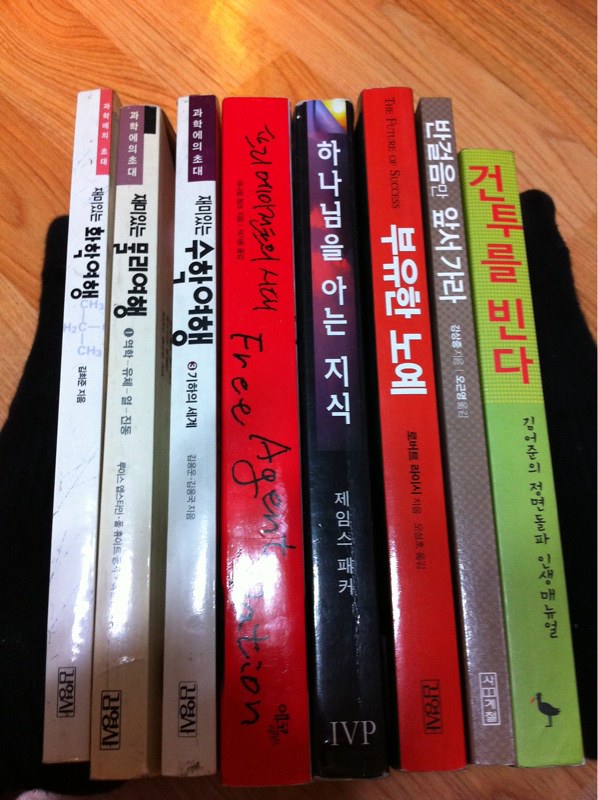This photograph captures a top-down view of eight paperback books meticulously lined up with their spines facing upward. The books are positioned on a wooden laminate floor, with a bright flash illuminating the scene from the bottom of the photo. Each spine displays titles written predominantly in Korean, except for one red book, the fourth in the lineup, which also features the English phrase "Free Agent Nation," seemingly handwritten. The books' spines vary in color and design: 

1. White with a red indent.
2. White with a purple indent.
3. White with a darker purple indent.
4. Solid red.
5. Black with sections in purple, orange, yellow, and blue.
6. Solid red.
7. Checkered grey.
8. Green with two shades, light and dark.

While the exact support holding the books isn't clear, it might be gloved hands or socked feet, possibly pressing the books together from either side to achieve the neat alignment for the photograph.